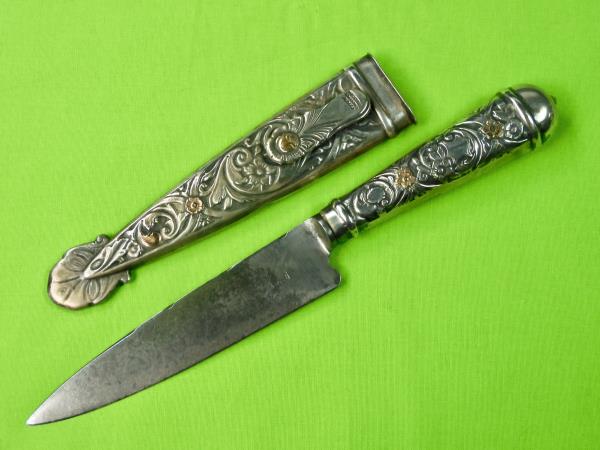This photograph showcases an intricately designed knife paired with its matching sheath, laying diagonally against a lime green backdrop, likely paper. The knife features a sharp, stainless steel blade, typical of a carving knife, while its handle is adorned with ornate metallic designs, incorporating both silver and subtle gold embellishments. The matching sheath, positioned above the knife, mirrors the handle’s elaborate design and color scheme, culminating in a distinctive metal leaf decoration at its pointed tip. Both the knife and sheath are displayed at a diagonal angle, emphasizing their craftsmanship and making their detailed designs stand out vividly against the vibrant background.